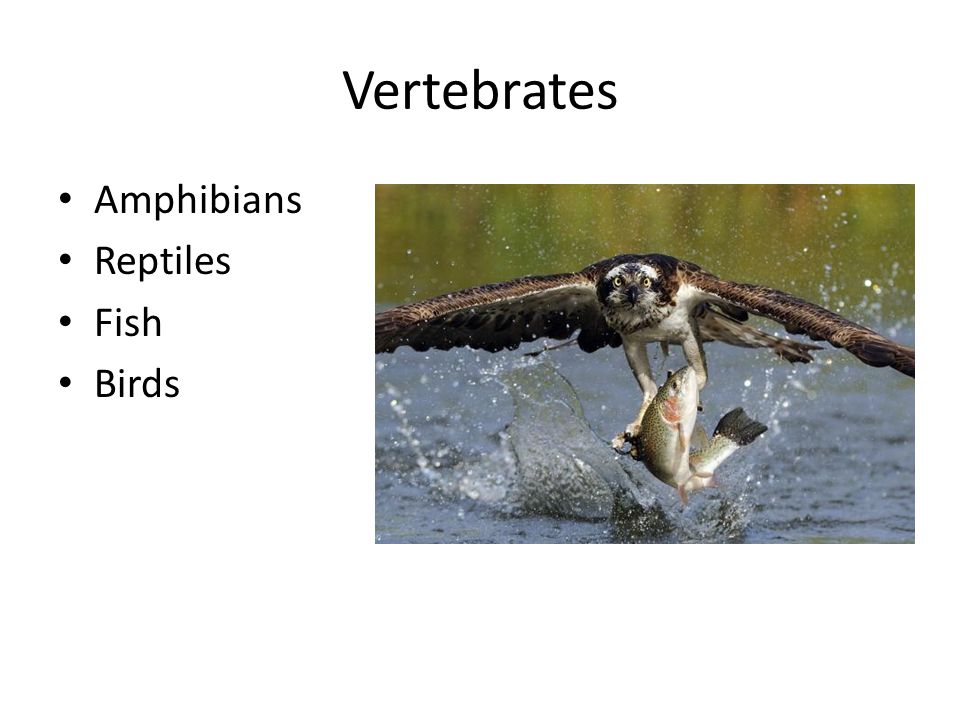The image is a detailed snapshot from a slideshow or presentation with a title at the top that reads "Vertebrates" in black font. On the left-hand side, there are four bullet points, each marked with a large dot. These points list "amphibians," "reptiles," "fish," and "birds." Occupying the right-hand side is an action photograph capturing an eagle in mid-flight, swooping close to a blue water surface to grab a silver fish with its talons. The fish is flapping vigorously, causing water to splash dramatically. The eagle, exhibiting a full wingspan, has a white head, yellow eyes, and brown feathers. The background above the water is a blurred green, suggesting grass or foliage in the distance. The photograph is approximately 4 inches wide by 3 inches tall.